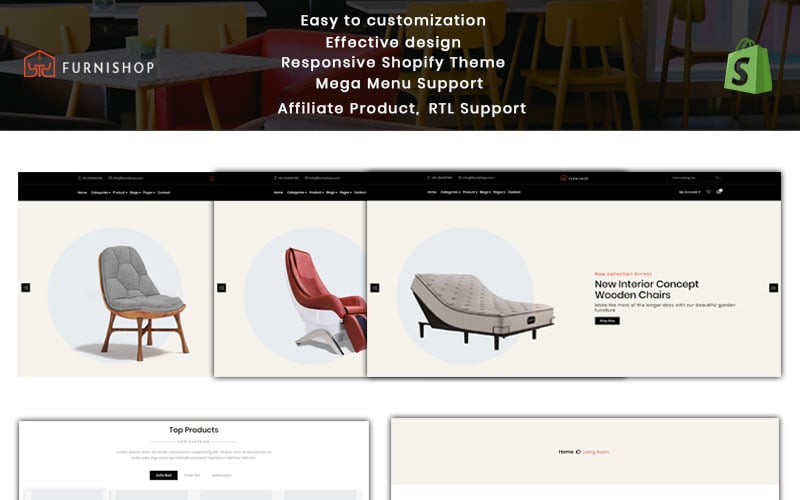This image is from a web page featuring the Furnishop brand. At the top of the page is a black navigation bar with a hazy overlay. On the left side of the bar is a red logo, which resembles a vertical bar, followed by the brand name "Furnishop" in white text.

In the center of the page, also in white text, are several phrases stacked vertically:
1. "Easy to Customization"
2. "Effective Design"
3. "Responsive Shopify Theme"
4. "Mega Menu Support"
5. "Affiliate Product, RTL Support"

On the right side of the bar is a green shopping bag icon with a black 'S' facing to the left.

The background of the bar features an image of several tables set with yellow and red chairs. Below this banner section is a section against a white backdrop containing a black bar with small white text that is illegible.

Following this, there are three horizontally aligned boxes:
1. The first white box features a bluish circle with a blue chair that has no arms and a gray cushion within it.
2. The second box displays a red, futuristic-looking reclining chair without arms, set on a white base.
3. The third, slightly longer box contains an image of a white mattress on a black frame, designed to allow the head section to be elevated. Beside it in black text is written "New Interior Concept," followed by "wooden chairs" and some additional black text that is illegible.

Below these boxes is a white eggshell section divided into two parts:
1. The left section, labeled "Top Products" at the top center in black text, has several rows of black text that are too small to discern, followed by a black bar with white text on the left.
2. The right section, more eggshell in color, features black text at the top center and red text beneath it, both of which are illegible. This section is partially cut off, revealing only the top portion.